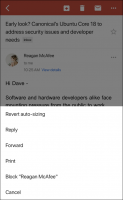In the image, we see two predominantly square sections that are somewhat blurry. The upper section features a red header containing several icons: a box with a red cross, a trash can, and a male symbol. Adjacent to these icons are three horizontally aligned dots. Directly below this header, there appears to be a comment section, although the text is exceedingly difficult to discern, rendered in light gray. 

The lower square contains a white box with various elements: faint and blurred text that seems to mention "revert" and "sizing," followed by indistinct icons for forwarding and printing. At the bottom of this section is a button labeled "Cancel," though it is similarly hard to read due to the overall blurriness of the image. Overall, the image has a substantial amount of illegible text and icons, making it challenging to interpret.